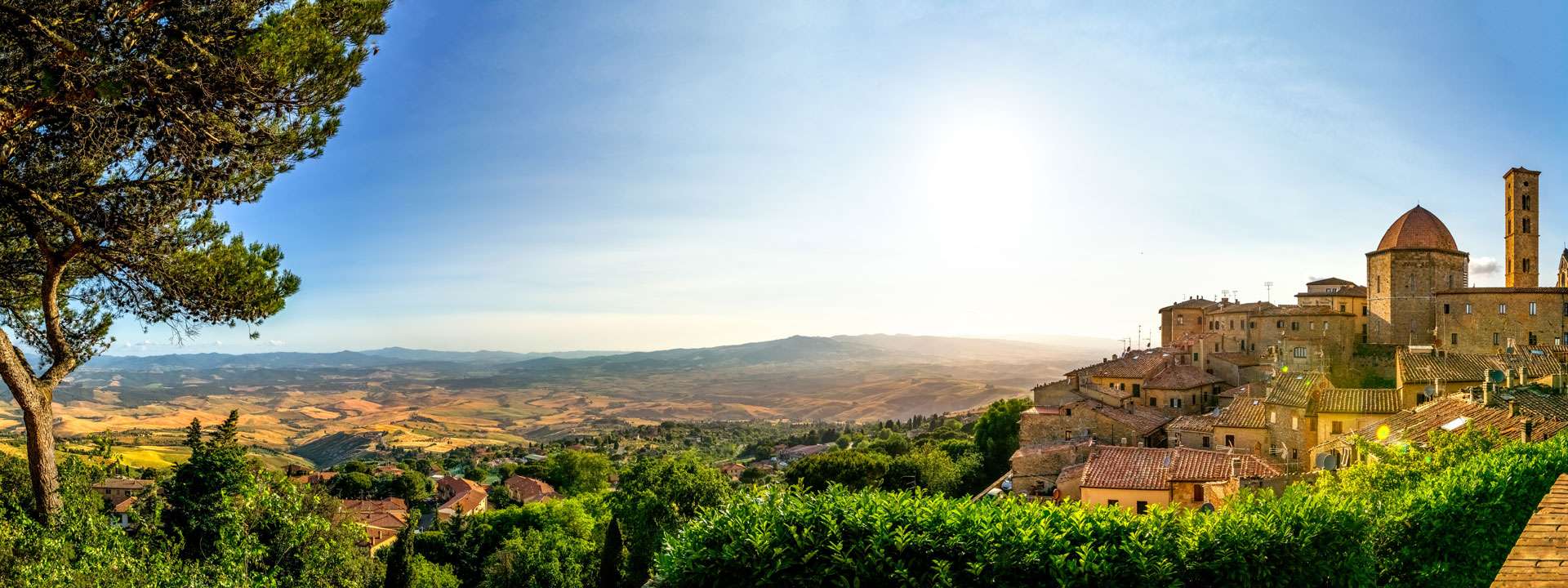This is a stunning wide-lens photograph with an exceptional level of clarity, capturing a picturesque landscape that seems almost photorealistic. To the right, there is an enchanting old-fashioned town with stone architecture and terracotta roofs, evocative of Spanish or Islamic style, possibly suggesting a location like Barcelona or somewhere in Portugal. Among the buildings, notable features include a distinctive copper dome roof and a tall rectangular tower that rises prominently above the rest.

The town is gracefully nestled on a hilltop surrounded by lush green foliage and scattered trees, harmonizing beautifully with the natural landscape. Below the town, the terrain transitions into neat lines of hedges or terraces, possibly used for crops. Extending into the distance, the land unfolds into slightly rolling hills and vast meadows in various shades of green and brown, indicative of a diverse and expansive countryside.

The sky above is a captivating bright blue, with a strikingly radiant white sun at its center, symbolizing bright daylight in one description and perhaps a bright white afterglow of sunset in another. A solitary tree stands out on the left edge of the image, framing the scene and adding to the photograph's serene composition. No clouds are visible, further emphasizing the clarity and tranquility of this exquisite landscape capture.